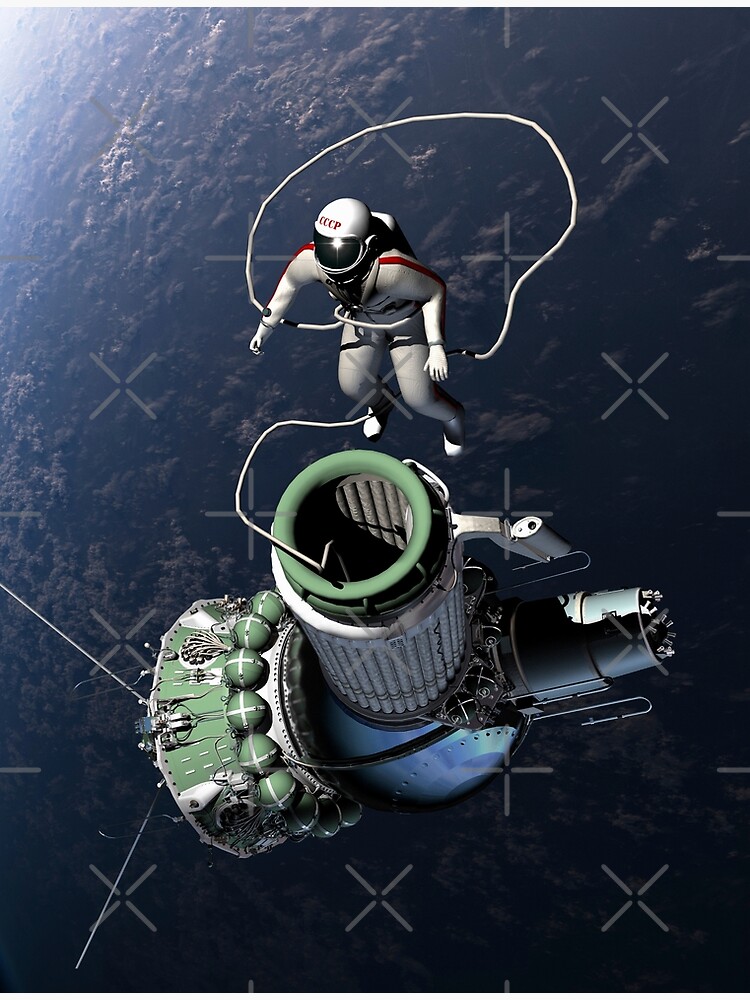In this highly detailed, photorealistic image, an astronaut is shown tethered to a satellite, seemingly floating above Earth. The astronaut is dressed in a predominantly white suit, accented with two red stripes running from the shoulders toward the elbows and red markings on the helmet that spell out "CCCP" above the visor. The helmet and suit both exhibit a high level of detail, contributing to the realism of the image.

A long tube or tether, which is green at the connecting end, attaches the astronaut to a round, silver satellite adorned with green accents and mechanical features. The tube seems to lead directly to an opening on the satellite that resembles a funnel shape, which might suggest an engine. This engine-like part is interspersed with wires and nine spherical objects wrapped around its base, adding a layer of complexity and intricacy.

The satellite itself features various protruding components, including an arm-like structure and a part with a saw-tooth design. One side of the satellite exhibits elements that are metallic and gunmetal-colored, adding depth and realism to the scene. In the background, a dark, cloudy planet—presumably Earth—is visible. The image hints at details like a faint outline of trees and a deep blue atmosphere, enhancing the sense of being suspended in the vastness of space.